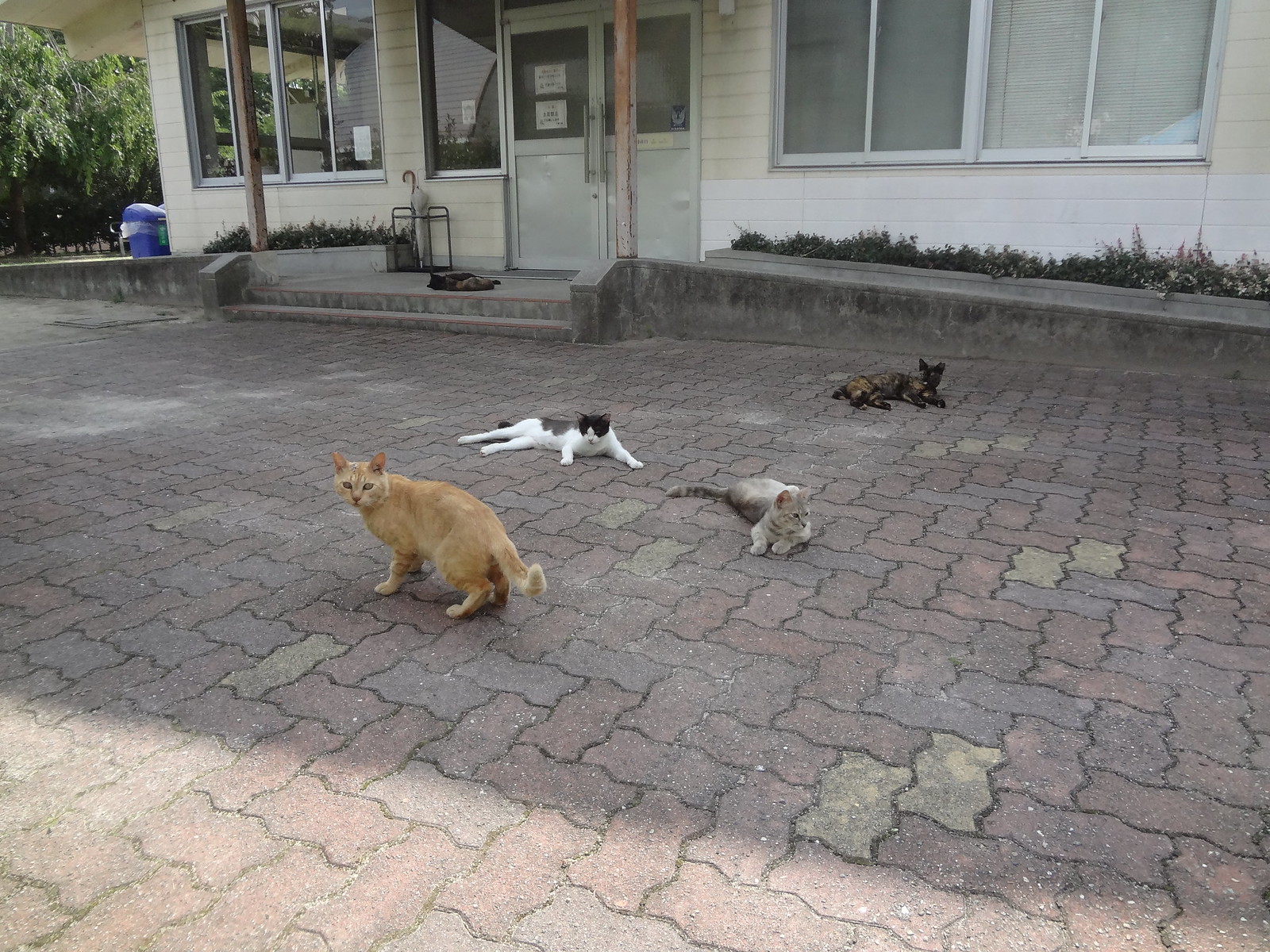This daytime outdoor photograph captures four cats lounging on a wavy reddish brick ground. The scene is set in front of a one-story building, likely a shop or community center, distinguished by yellow vertical boards, numerous windows, and double doors adorned with business-style handles and posted notices. A variety of lush, green trees, and tall, shaggy bushes frame the left side of the background. Concrete ramps flank either side of a small porch step leading to the entrance, with an umbrella rack visible, as well as a blue recycling bin around the building's corner. The foreground features an orange cat turning its head toward the camera, providing a side view of its body and a front view of its face. Next to it, a gray cat lays down with its head turned to the side. On the left, a white and gray cat reclines on the ground, while a speckled rusty brown and black cat rests with its paws extended forward in the far background. The overall atmosphere is shaded, suggesting a sunny day.